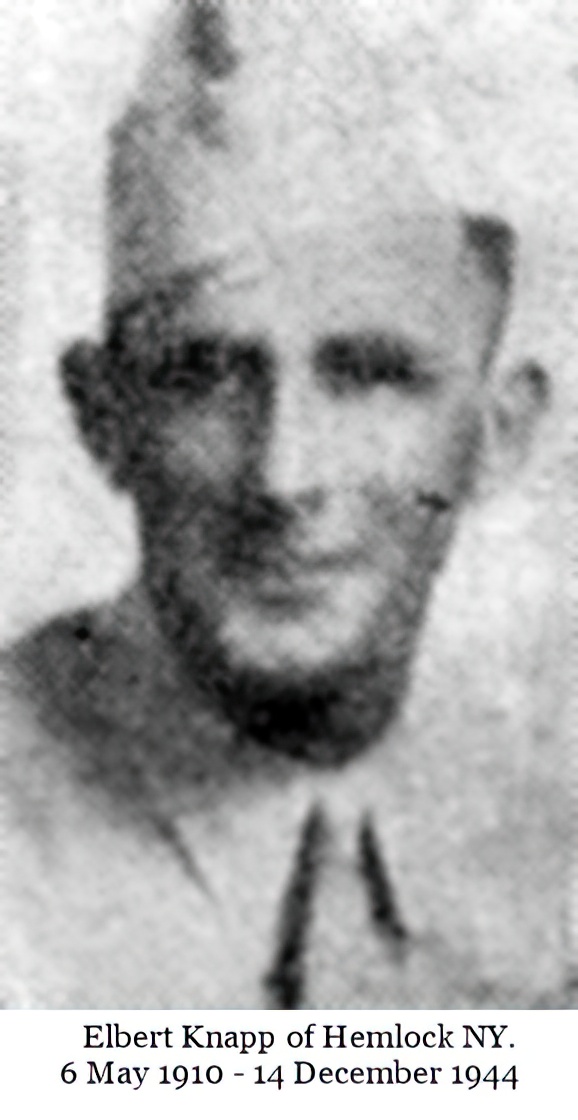This is a black and white vintage photo of Albert Knapp from Hemlock, New York, born on May 6, 1910, and died on December 14, 1944. The image, scanned with very few pixels, reveals a grainy and fuzzy quality that suggests its age. Albert, a white male with a thin, long face, is dressed in what appears to be a military or naval dress uniform, including a light-colored button-down collared shirt, a tie, and a triangular-shaped service hat tilted to the side. His typical short army haircut and lack of facial hair are noticeable, as are his slightly protruding ears. Taken in a neutral background, likely at a photo studio, this image commemorates Albert Knapp's service, as he possibly died during World War II.